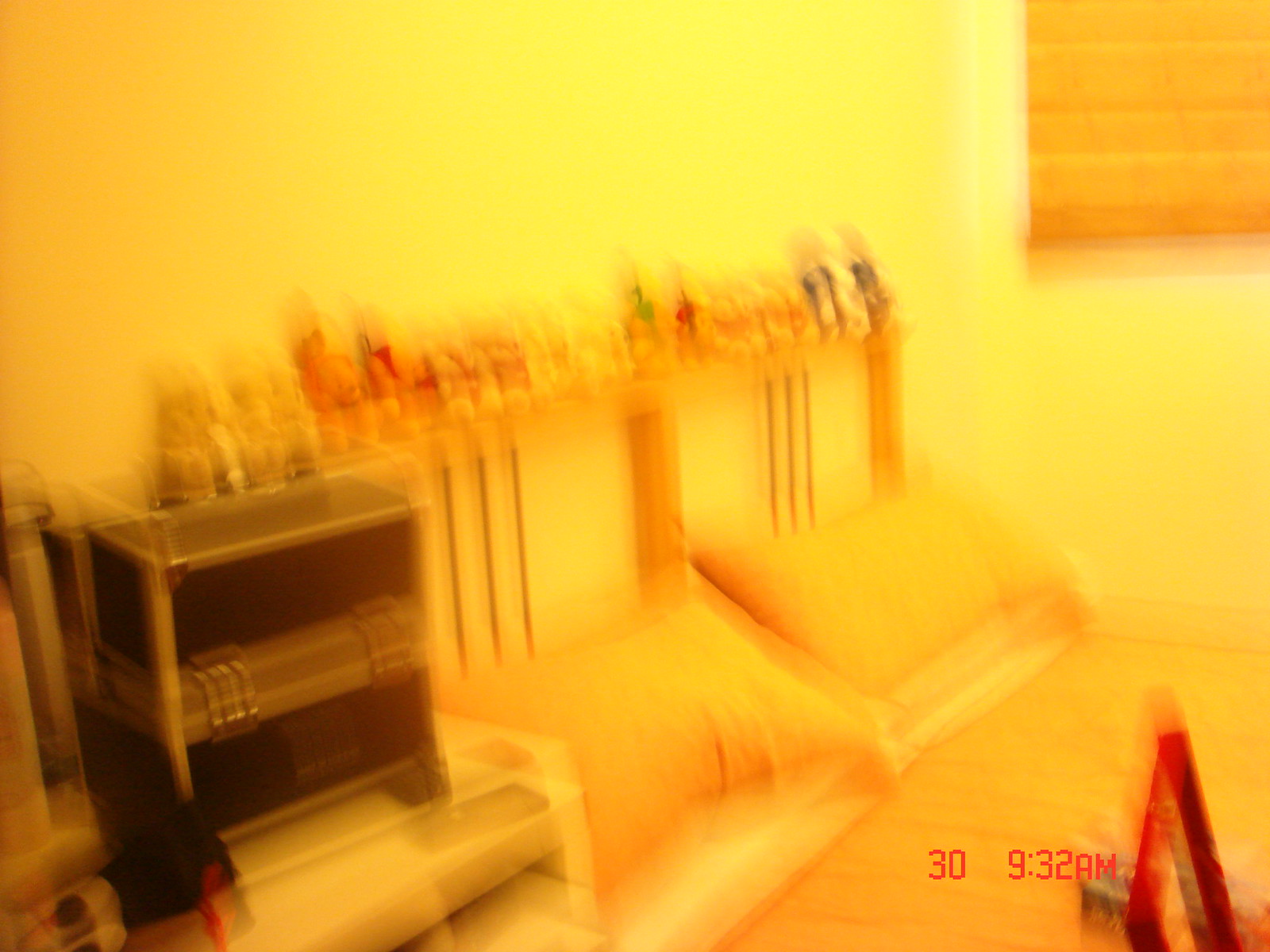This photograph, though blurry, captures a cluttered bedroom scene with a warm yellow hue, likely due to the ambient lighting. The bed is the focal point, featuring a frame crowded with small toys and knick-knacks that cover it from end to end. The room has a window draped with a thin paper covering acting as makeshift blinds. A small musician's equipment box can be seen nearby, contrasting with the larger items. Two pillows rest on the bed, and an easel is also visible in the space, suggesting an artistic atmosphere. The timestamp on the image shows 9:30 a.m., indicating the time this cozy, albeit cluttered, bedroom scene was captured.